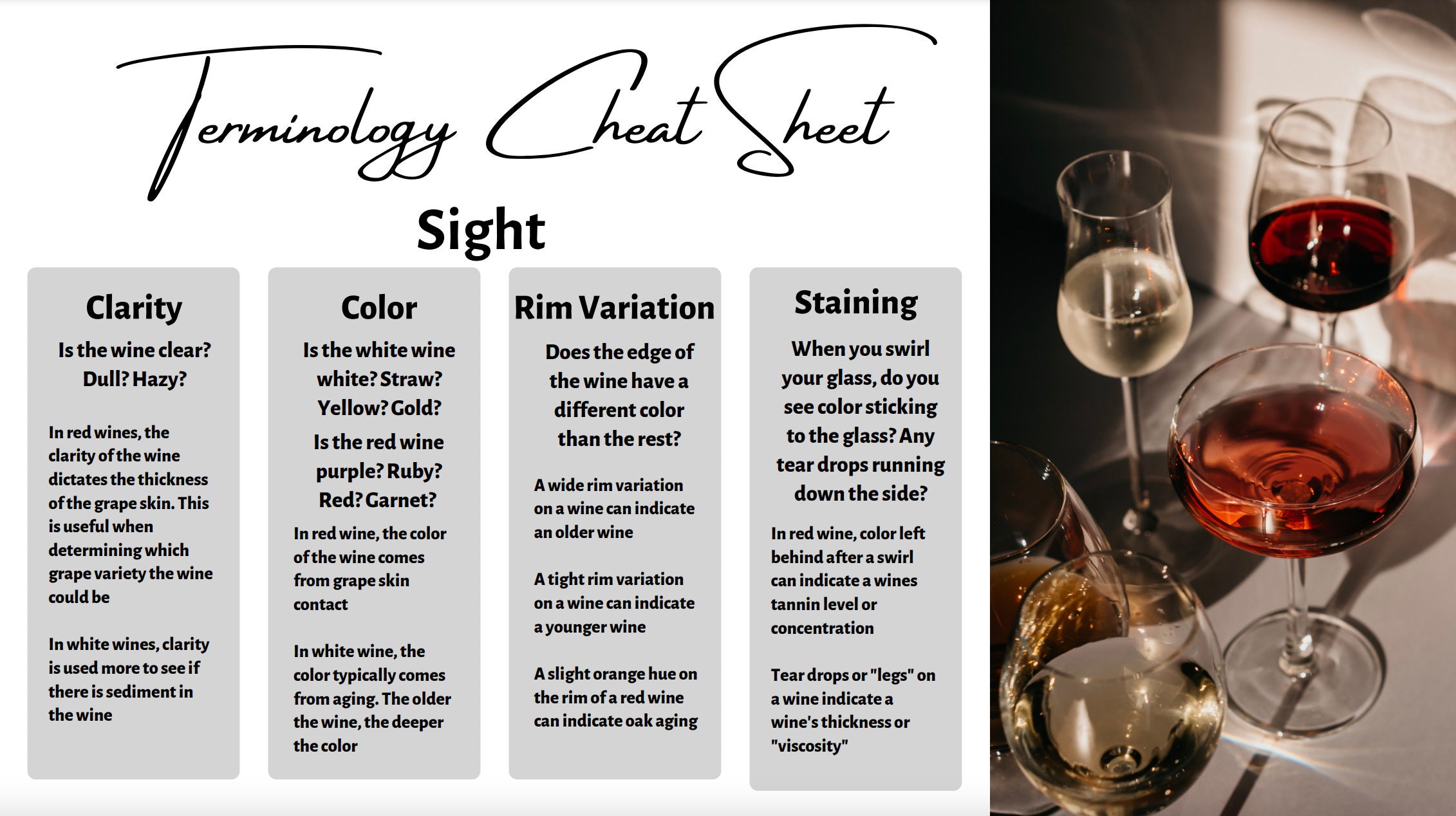The image is a horizontally rectangular guide for wine tasting with a pristine white background. Centered at the top in black cursive text is the title "Terminology Cheat Sheet." Beneath this, the word "Sight" introduces a detailed chart divided into four vertical gray rectangles, each describing different aspects of wine observation. The first rectangle, labeled "Clarity," poses the question: "Is the wine clear, dull, hazy?" followed by two paragraphs explaining how clarity in red wines indicates the thickness of the grape skin and in white wines helps detect sediment. The second rectangle, titled "Color," prompts viewers to assess whether the wine is white, straw, yellow, or gold, and if the red wine is purple, ruby, red, or garnet, plus an additional two paragraphs expanding on this. The third rectangle covers "Rim Variation," asking if the edge of the wine differs in color from the rest, elaborated upon in three paragraphs. The final rectangle, "Staining," inquires if swirling the glass results in colors sticking to the glass or teardrops running down the sides, with two supporting paragraphs explaining this phenomenon. 

To the right of the chart is a color image featuring five wine glasses of different shapes and sizes, containing wines in various hues from almost clear to golden, light red, and dark red. The arrangement includes two glasses in the back—one slender with white wine and the other thicker with red wine. In the front, a wider, shorter glass filled with a lighter red wine is positioned center-right, while two more glasses with white wine are situated towards the left side of the picture. The overall composition provides a comprehensive visual and textual guide to the visual assessment of wine.